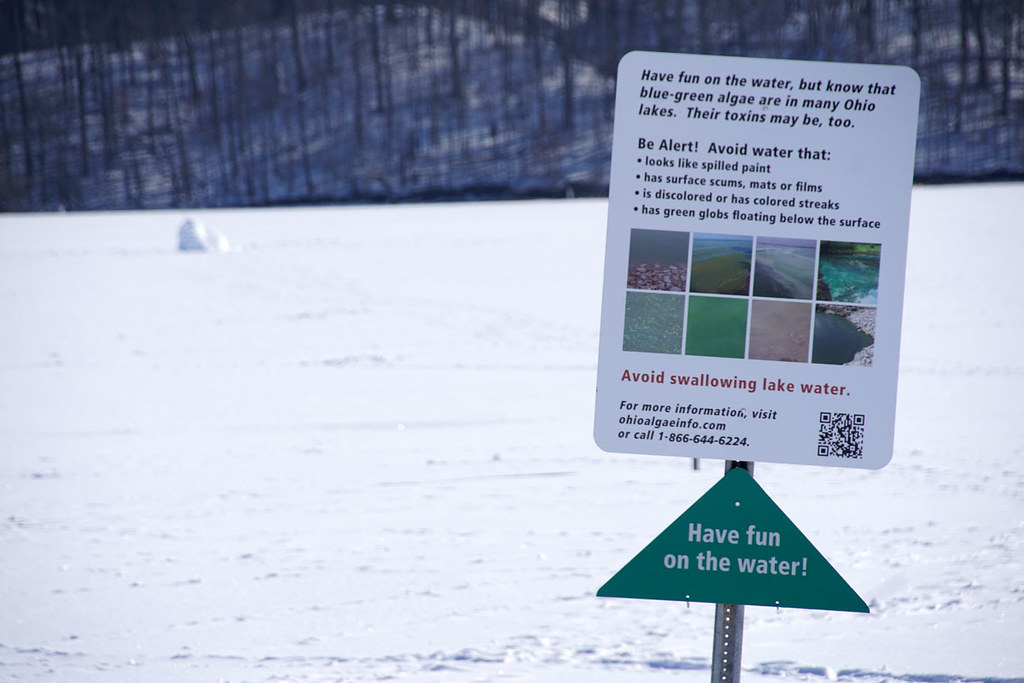The photograph captures a stark winter landscape with a snow-covered, frozen lake in the foreground and distant hills dotted with bare tree trunks. Dominating the scene is a large sign planted in the snowy ground. The sign, predominantly white with black text, prominently reads, "Have fun on the water, but know that blue-green algae are in many Ohio lakes. Their toxins may be, too. Be alert." It warns to "Avoid water that looks like spilled paint, has surface scums, mats or films, is discolored or has colored streaks, and has green globs floating below the surface." Additionally, it advises against swallowing lake water. The sign also includes eight illustrative images depicting the hazardous conditions described. For more information, it directs viewers to visit OhioAlgaeInfo.com or call 1-866-644-6224, emphasizing ease of access with a QR code at the bottom right. Below these warnings, a green triangle with white lettering uplifts the mood slightly with the message, "Have fun on the water." The chilling yet informative display stands as a stark reminder amidst the serene, snowy backdrop of Ohio’s winter landscape.